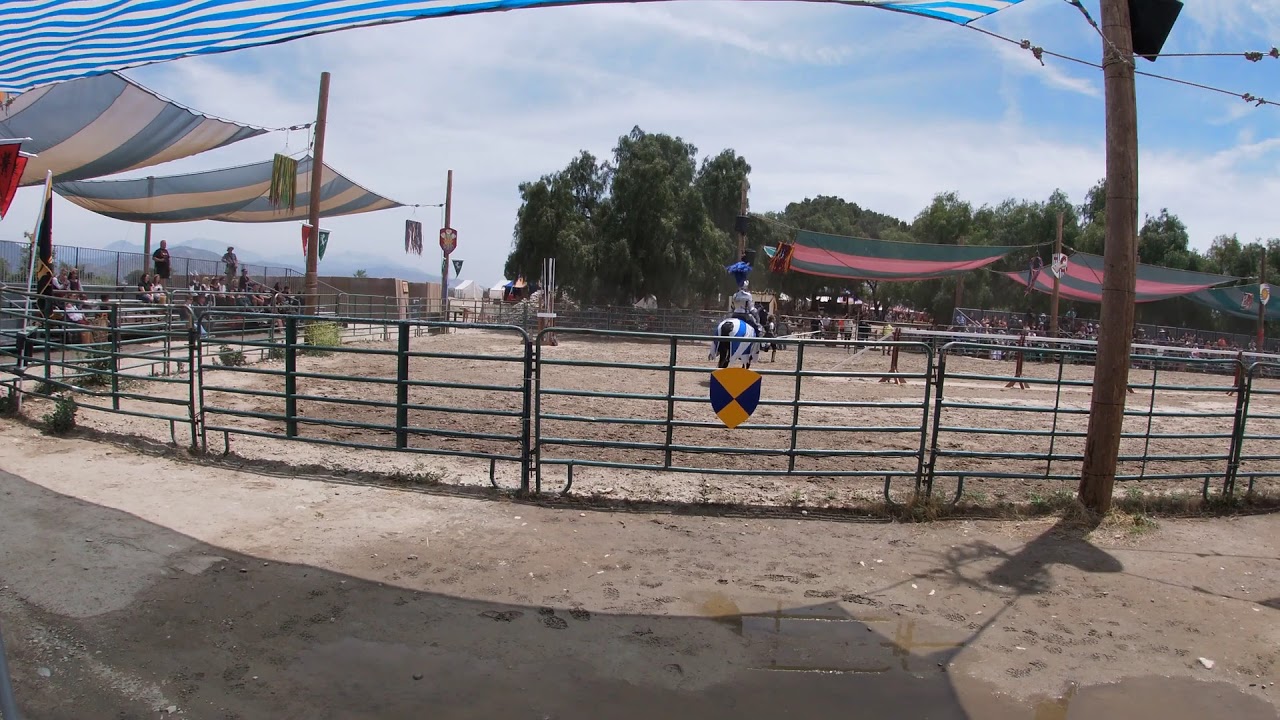The photograph captures a vibrant scene at a Renaissance fair during a jousting event in a large, corralled horse-riding arena. Dominating the center of the image is a rider in full knight regalia, mounted on a horse draped with a blue and white striped blanket, indicative of the blue team. The arena's sandy and slightly muddy ground bears the footprints of numerous fairgoers, adding to the lively atmosphere. Surrounding the arena are metal corral gates and telephone pole-like posts, adorned with shading banners and team colors. 

Blue and white striped awnings cover several sets of bleachers on both sides of the corral, which are populated by spectators. The blue team's bleachers are about a third full, while the red team's section is nearly at capacity, highlighting the event's popularity. In the background, behind additional awnings, a line of trees stretches out under a clear, blue sky with only a few white clouds. Overall, the scene is a bustling, picturesque snapshot of a thrilling Renaissance fair jousting tournament on a clear day.